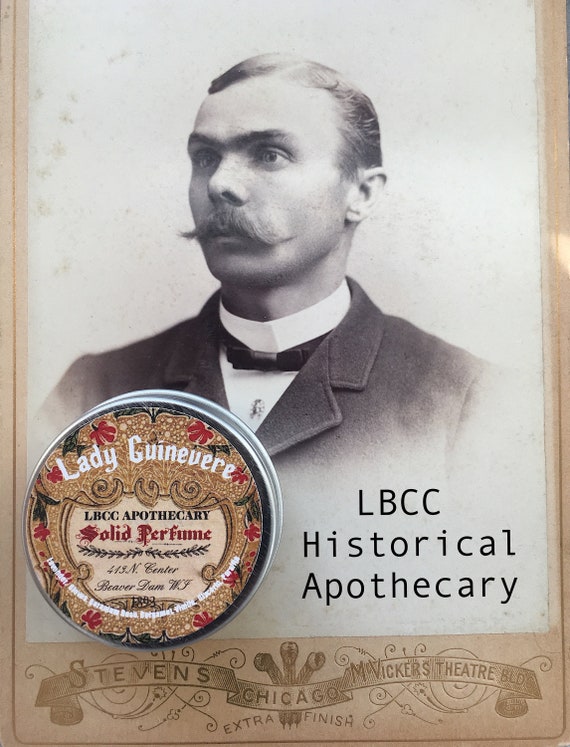This detailed image depicts an old, black and white photograph of a man with slicked-back, thinning hair, and a prominent handlebar mustache. He is dressed in a basic cotton-looking suit with a white-collared shirt and a small black bow tie, giving the appearance of a relaxed, contemplative stare off to the left. The photograph is part of a card bordered in a delicate, light gold hue, particularly on the left, right, and bottom edges.

Overlaying the bottom left of the card is an ornate tin canister, adorned with a gold leaf print and red floral designs interspersed with intricate small brown swirls and dots. The canister is marked with the text "Lady Guinevere, LBCC Apothecary, Solid Perfume, 413 N Center, Beaver Dam, WI, 1893." Adjacent to this, the text "LBCC Historical Apothecary" is clearly printed in black. Below this setup, on a tan banner at the bottom of the image, it reads "Stevens, Chicago, McVicker’s Theater Boulevard, Extra Finish," emphasizing the card’s historic and decorative authenticity.